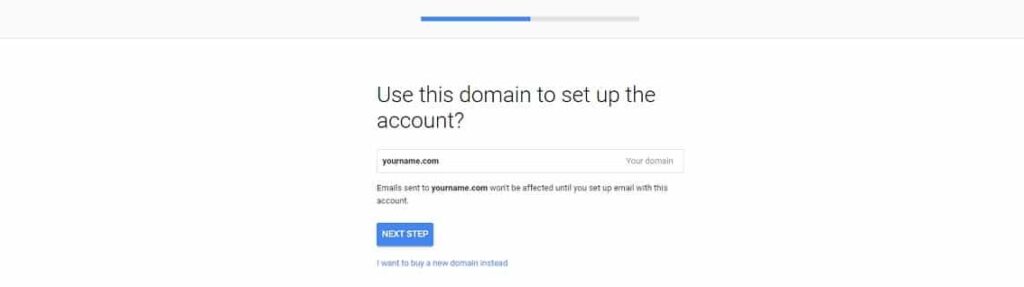The image depicts a setup screen for a company's account registration process. The interface features a prominent gray bar spanning the entire width of the computer screen. Within this bar, centrally located, is a smaller bar that is half blue and half gray. Below this bar, a question is displayed: "Use this domain to set up the account?" Directly beneath this question, the placeholder text "yourname.com" is shown, followed by faint and barely readable text that potentially says "your domain."

Further down, another line of text states: "Email sent to yourname.com, support the affected until you set up email with the account." A prominent "Next Step" button in a blue box is situated below this information. There is additional text beneath the blue box, but it is illegible due to its minuscule size. The overall design is minimalist and straightforward, suggesting this is likely one page within a multi-step registration process.